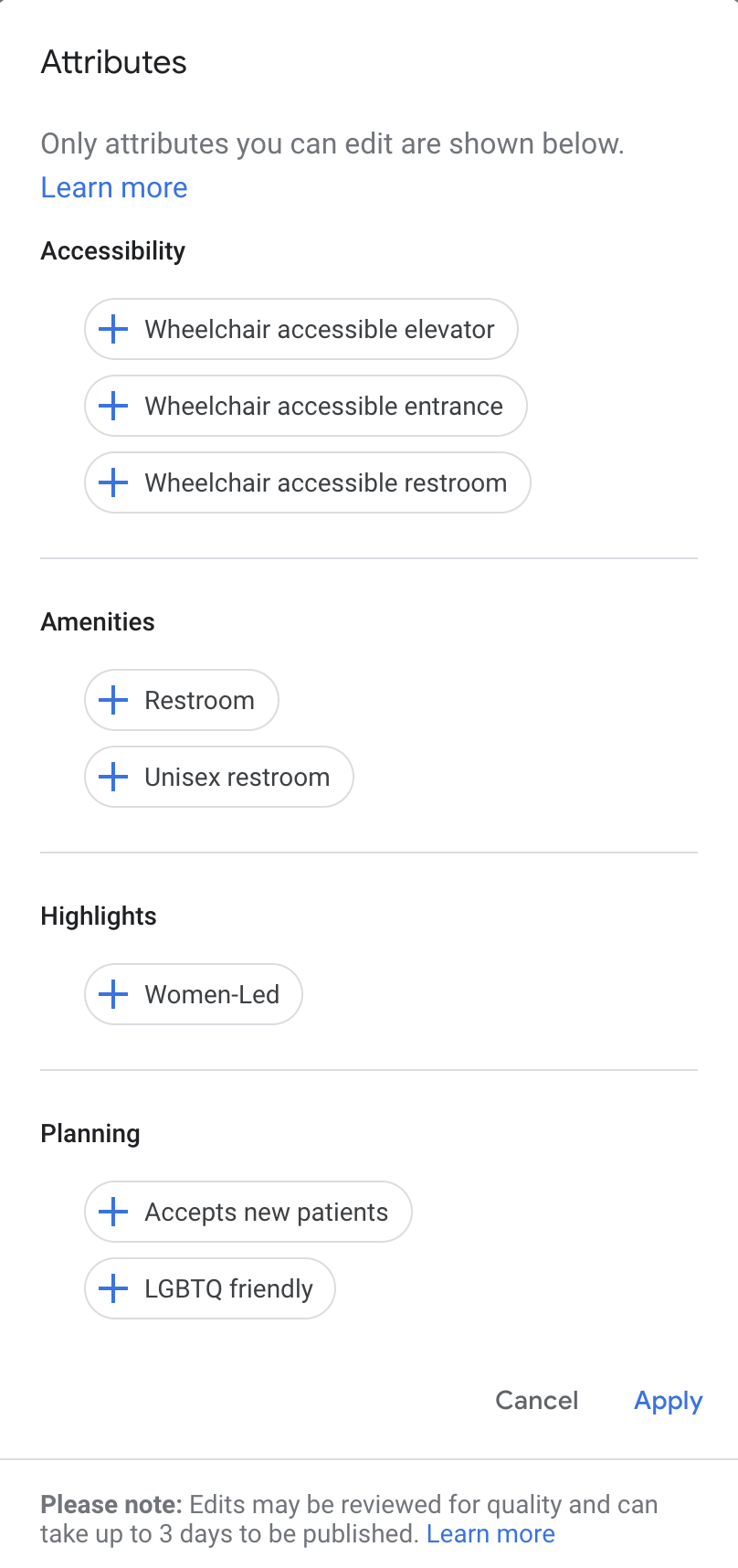This image is a detailed amenities and features page for a specific location. At the top left, there is a section labeled "Attributes" in black text, followed by a gray note stating "Only attributes you can edit are shown." Below that, there is a hyperlink "Learn more" also in gray text.

The first primary section under the "Attributes" header is "Accessibility," which includes:
- Wheelchair accessible elevator
- Wheelchair accessible entrance
- Wheelchair accessible restroom

Each of these accessibility features is preceded by a blue plus sign enclosed in an elliptical shape, and they are separated by a gray horizontal line.

Moving downward, the next section is titled "Amenities" in black text. This section lists two options:
- Restroom
- Unisex restroom

Both options are capitalized at the beginning and have a blue plus sign to their left, each enclosed in a gray elliptical shape. Another gray horizontal line separates this section from the next.

Following that is the "Highlights" section, also in black text. It includes a single listing:
- Woman-led

This is indicated by a blue plus sign and is separated by the same gray horizontal line.

Finally, the "Planning" section appears in black text, listing:
- Exceptionally patient
- LGBTQ friendly

Both features are aligned with blue plus signs next to them. 

At the bottom of the page, there is a gray "Cancel" button to the right and a blue "Apply" button. Following is a disclaimer that starts with "Please note" in bold, stating: "Edits may be reviewed for quality and can take up to three days to be published," with a "Learn more" hyperlink in blue text to the right.